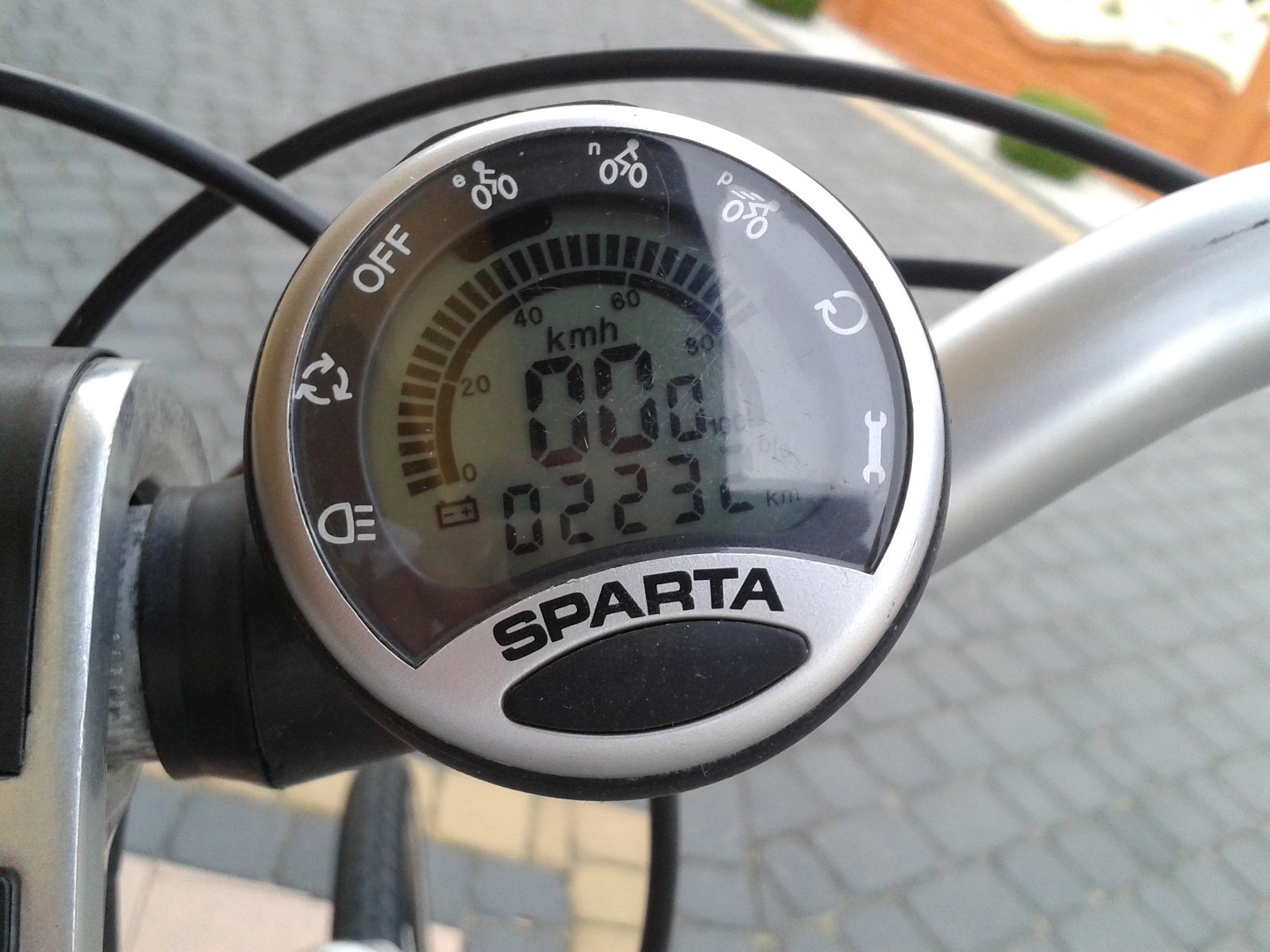A close-up photograph taken outdoors showcases a bike speedometer. The central feature of the image is the speedometer dial, prominently displaying the text "km/h" (kilometers per hour) in white on a black background. The speedometer reads zero, indicating the bike is stationary. Below this, an odometer shows the digits "02232," which might represent the cumulative distance traveled.

The speedometer itself is encased in a frame that is predominantly gray and black, with the face and inner components presenting a darker gray hue under a clear lens. To the left of the dial, there is a small battery icon, indicating the device’s power status through the symbols for positive and negative.

Surrounding the lens on its perimeter, there are various symbols, including a white light icon and what appears to be a symbol to toggle the device on and off. Along the top edge of the dial, small bicycle-related icons are arranged, further confirming the device's purpose.

The right side of the image features a portion of the bike’s handlebar, made from brushed metal and black rubber components. Gear cables, appearing to be of heavy-duty design, extend from the central frame, which is also a mix of brushed metal and rubber materials. The background suggests the bike is situated on a gray, patio-like surface, adding an outdoor and active feel to the scene.